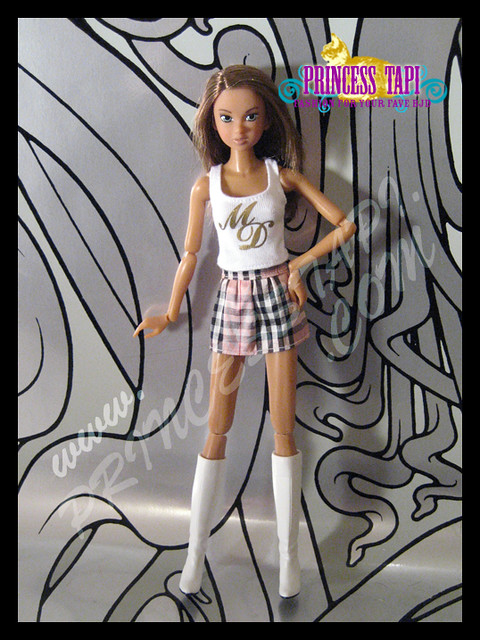The image features an advertisement showcasing a doll named Princess Tappy, prominently positioned in the center of the frame. This doll, resembling a Barbie in style but unique in its branding, sports flowing brunette hair and bright blue eyes, complementing her cheerful smile. Her pose is dynamic: the left arm rests confidently on her hip while the right arm is uplifted towards the right-hand side. Princess Tappy is dressed in a chic outfit comprising of a white tank top emblazoned with the cursive letters "ML," paired with a short, plaid skirt, and knee-high white boots. Above her head, bold pink text on an orange background announces "Princess Tappy," accented by whimsical light blue spirals. The backdrop behind the doll is a psychedelic design featuring various colors such as black, gray, white, off-white, different shades of yellow, purple, light blue, brown, pink, and some gray shapes, providing a vibrant and eye-catching contrast. A black border encloses the entire image, adding a polished finish to this striking advertisement for Princess Tappy's fashion-forward appeal.